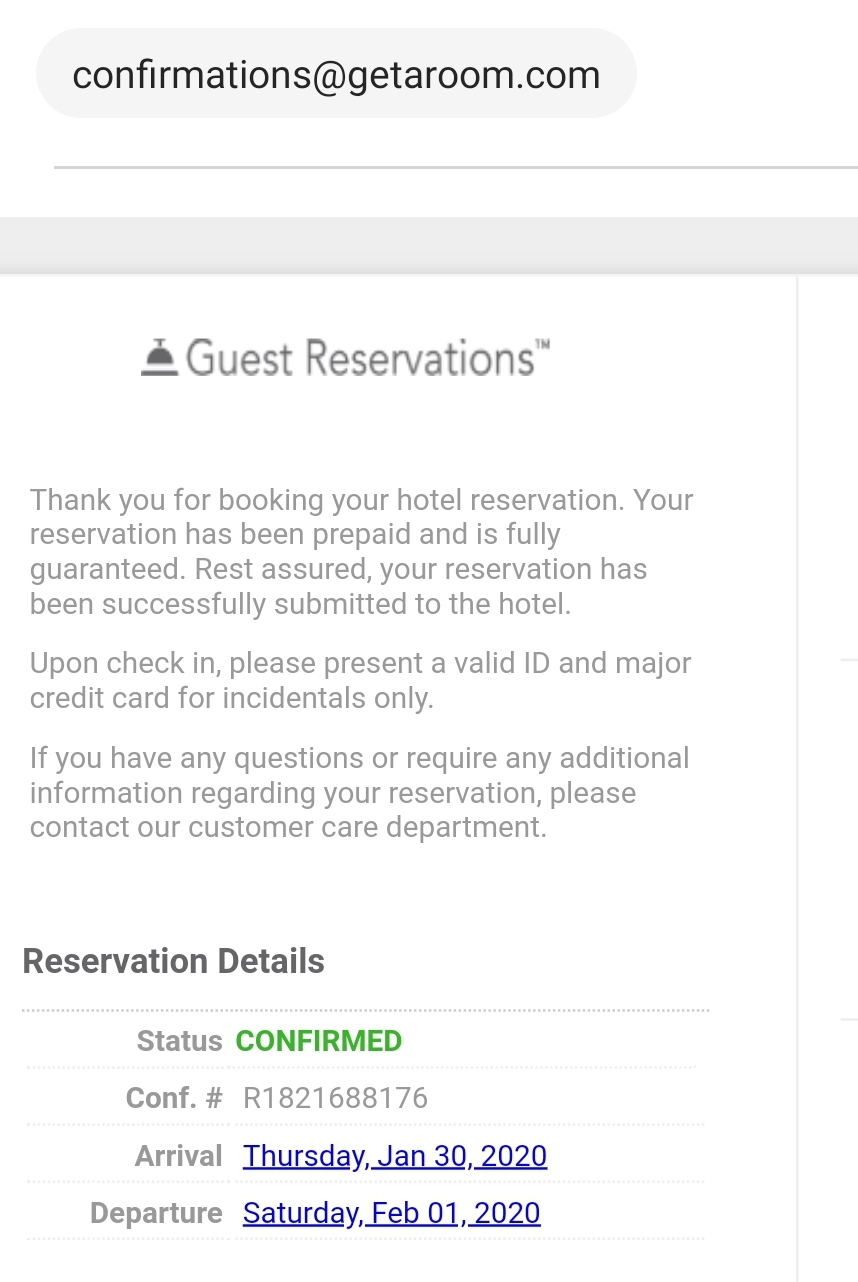This image is a screenshot from a booking confirmation email sent by confirmations@getaroom.com. At the top, the email address is prominently displayed to indicate the sender. Below the email address, there's a grey bar with a bell icon typically seen at hotel front desks, alongside the text "Guest Reservations." 

The main body of the email expresses gratitude for the hotel reservation, reassuring the recipient that the reservation has been prepaid and fully guaranteed. It confirms that the booking details have been successfully submitted to the hotel. The email advises guests to present a valid ID and a major credit card for incidental expenses upon check-in. It also provides a point of contact for any questions or additional information through their customer care department.

In the section titled "Reservation Details," the status of the reservation is highlighted in green as "Confirmed." Below this, the confirmation number is listed as R1821688176, followed by the arrival and departure information:
- Arrival: Thursday, January 30th, 2020
- Departure: Saturday, February 1st, 2020

The dates of arrival and departure are in blue and appear underlined, indicating that they might be clickable links for additional options or details.